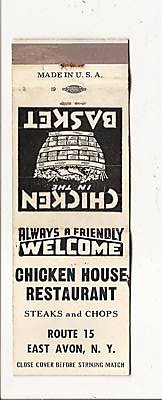The image depicts a vintage matchbook cover unfolded to reveal both sides, highlighting its weathered, yellowish paper. At the top, positioned horizontally, is the striking strip, rendered in gray. Beneath this strip, in small black letters, it reads "Made in USA." The back cover of the matchbook, shown upside down, features a black square with white text that says "Chicken in the Basket," accompanied by an illustration of an upside-down basket. The front cover, displayed right-side up, includes the welcoming words "Always a Friendly Welcome," followed by "Chicken House Restaurant," "Steaks and Chops," and "Route 15, East Avon, New York." The bottom of this cover carries the instruction, "Close Cover Before Striking Match." The entire matchbook, captured in a close-up photograph, exudes a nostalgic charm with its black-and-white design and faded, vintage appearance, typical of mid-20th century printed collateral.